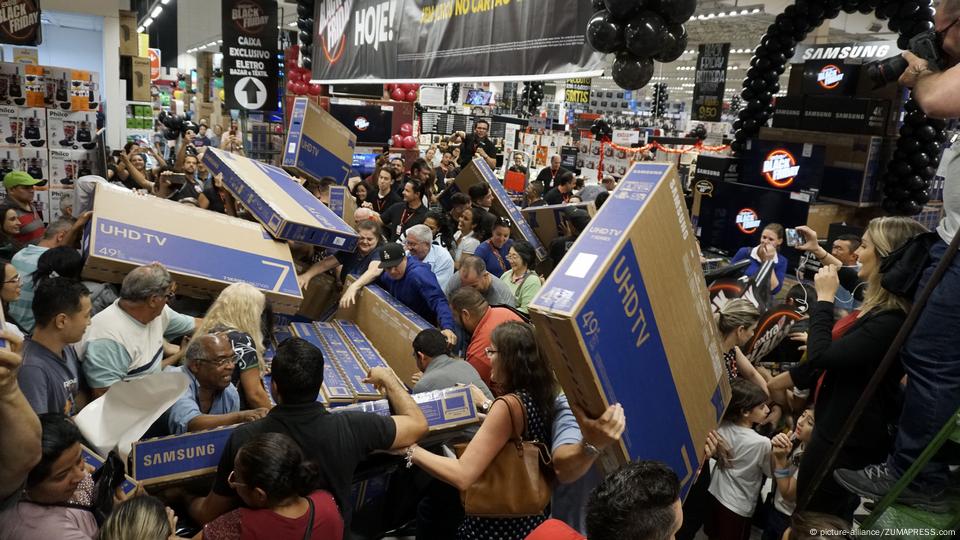This image captures a chaotic Black Friday sale scene inside a large electronics store, reminiscent of a Best Buy or Wal-Mart. The frenzy centers around 49-inch Samsung UHD TVs, identifiable by their brown boxes with prominent Samsung branding in white and a distinct blue rectangle indicating high-definition features. Shoppers are visibly fighting over these televisions, creating a tense atmosphere on the shop floor. A palette of these TVs appears to be the focal point of the scramble, with numerous people clutching the large boxes while others desperately reach for the remaining stock. Employees in the background look noticeably concerned as they witness the unruly behavior. The overall scene reflects a mix of panic and greed, with people standing over one another in their attempt to secure the heavily discounted TVs. The presence of balloons and store signage further supports the idea of a special sale event, adding to the frenzied mood.